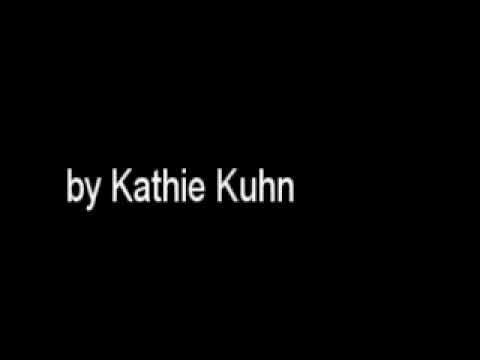This image depicts a solid black rectangular background, slightly longer than it is tall, with a simple yet striking white text in the center. The text, positioned centrally from top to bottom but left-justified horizontally, reads "BY Kathy Kuhn". The letters 'B-Y' are in small caps, followed by the full name 'Kathy Kuhn', with 'Kathy' spelled as K-A-T-H-I-E and 'Kuhn' spelled as K-U-H-N. The font is a sans serif style, resembling Arial Narrow. The overall impression is one of minimalist design, with no gradients or additional visuals, focusing solely on the text against the stark black background.